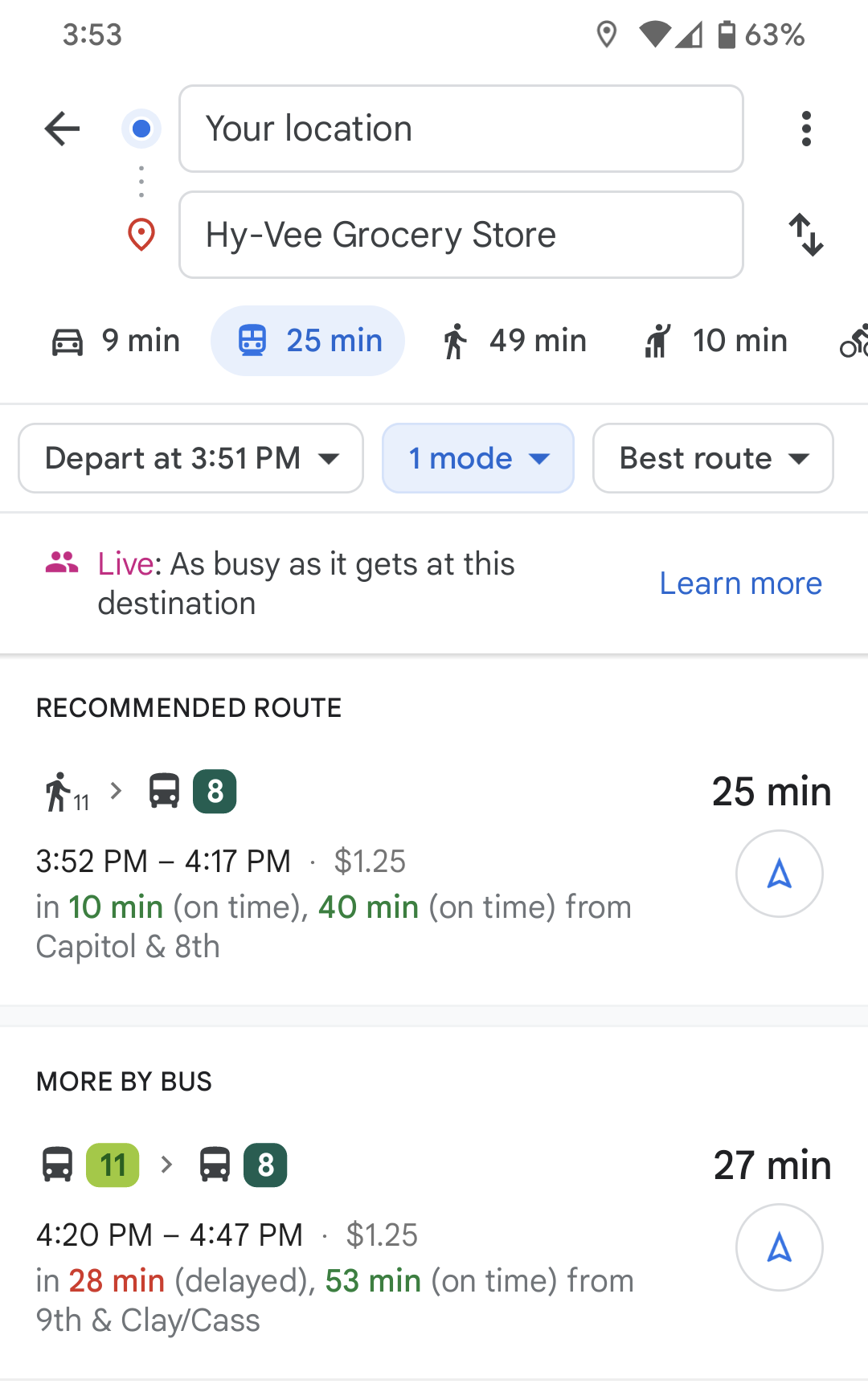The image is a detailed screenshot from the Google Maps transit section displayed on a white background. At the top of the image, the status bar information is visible, indicating location pin "353," a full Wi-Fi signal, three out of four bars of cellular service, and a battery life at 63%. 

Below the status bar are two text boxes: one labeled "Your location" accompanied by a blue dot on the left, and the other labeled "Hy-Vee Grocery Store" with a red pin on the left. Between these boxes, there is a back arrow on the left and a hamburger menu along with an up-down swap icon on the right, allowing users to interchange the starting point and destination.

Further down, there are icons representing various transportation modes: car, transit (highlighted in blue), walking, ridesharing, and biking. The respective travel times next to these icons are nine minutes for driving, 25 minutes for transit, 49 minutes for walking, and 10 minutes for ridesharing. 

The image includes details for departing at 3:51 PM. Below this, in blue text, it indicates "One mode" and "Best route" on the right. The "Live" status in pink suggests that the destination is as busy as it gets, with a black note indicating this status. To the right is a blue "Learn more" link.

The suggested transit plan is highlighted under "Recommended route," with directions to walk 11 minutes and then take the "8" bus, which is marked in green. An additional option under "More by bus" suggests taking the "11" bus, followed by a transfer to the "8" bus.